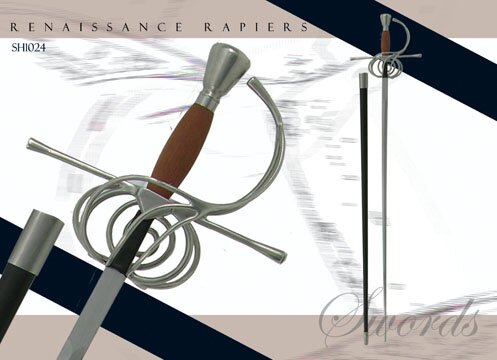The image is a detailed, ornate poster showcasing a Renaissance rapier. Dominating the right side of the image is a full-length view of the elegant rapier, which features a long, silver blade with a brown handle adorned with a swirl pattern and intricate silver details. Next to the rapier is a tall black sheath, capped with silver ends. The left side of the image displays a close-up of the handle, emphasizing the craftsmanship in the circular and spiral metal designs. The top left corner of the image bears the text "Renaissance Rapiers" in black against a light mauve banner. Similar mauve banners border the top and bottom of the image, intersected with diagonal black bands, adding a touch of elegance to the overall composition. In the bottom right corner, the word "swords" is written in a delicate script font. The background of the image is primarily white, ensuring that the details of the rapier and the accompanying elements stand out.